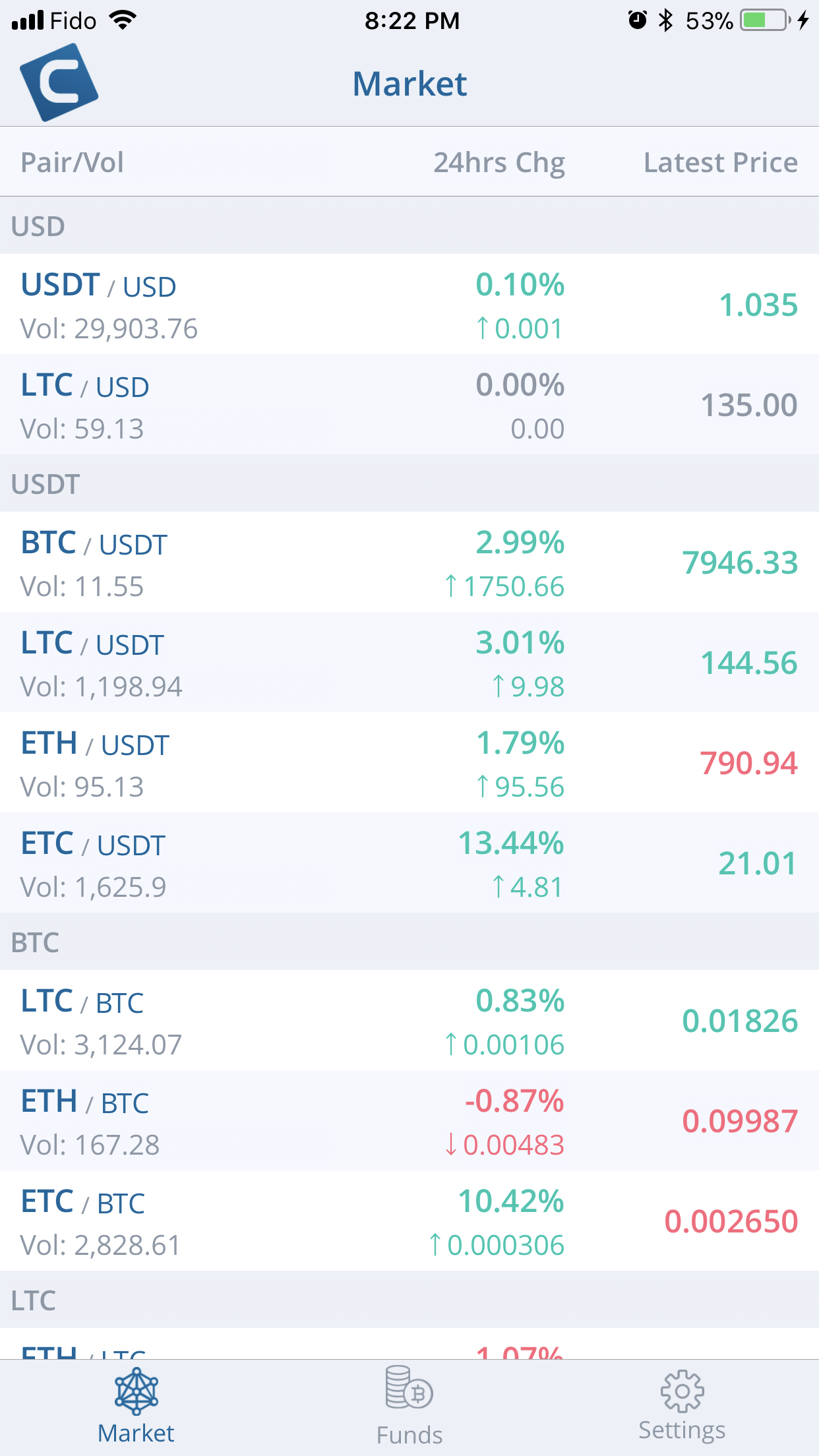In this detailed screenshot taken from a smartphone, the image captures various on-screen elements and icons. 

At the very top of the screen, the status bar displays several indicators. On the top right, the battery icon is shown with a lightning bolt, indicating that the phone is currently charging. To the left of the battery icon, the battery level reads at 53%. Adjacent to this is the Bluetooth icon followed by an alarm clock icon. Centering the top, the current time is displayed as 8:22 PM.

On the top left, the signal strength icon shows full bars next to the carrier name "FIDO" and a Wi-Fi icon, both indicating high connectivity.

Just below the status bar and slightly to the right, a logo appears that seems to be the letter 'C' within a tilted square, resembling a diamond shape. Below this, in the top middle, the word "Market" is prominently displayed in blue, suggesting this screenshot is taken from a financial or trading application.

Further down, various financial metrics and trading pairs are presented. On the far left vertically, a list reads "USD", followed by trading statistics such as "USDT/USD volume 29903.76." Also listed are trading pairs and currencies, including "USDT" and "BTC."

At the bottom of the screenshot, a navigation bar splits into three categories: "Market," "Funds," and "Settings," offering quick access options within the application.

This intricate snapshot is a detailed capture of a trading or financial monitoring app, emphasizing connectivity, real-time market details, and navigational features.